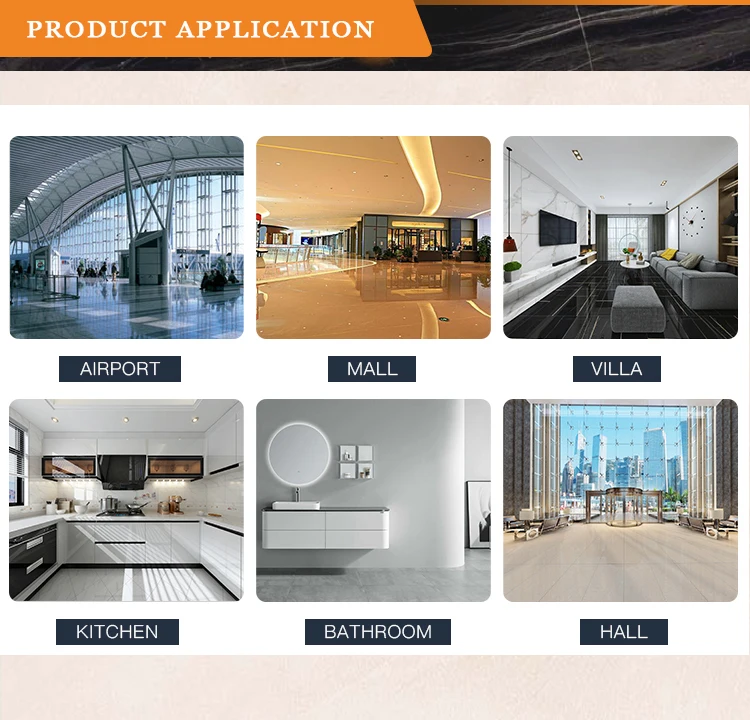Here's a detailed and cleaned-up caption for the image:

"This is a screenshot of a website, featuring a sophisticated design. At the top, there is a striking black-and-white marble banner. Positioned on the upper left side of this banner is an eye-catching orange rectangle with white text that reads 'Product Application.' Directly below the marble banner, there is a horizontal gray bar. Beneath this gray bar, the background turns white, showcasing two rows of three horizontally aligned photos, each carefully labeled. 

The first photo on the left is labeled 'Airport' and features a spacious airport waiting lobby with large, open windows that allow natural light to flood the area. In the center, there is a 'Mall' labeled photo, capturing the interior of a very modern  and futuristic mall filled with people standing outside a store. Finally, on the right, there's an image labeled 'Villa.' This photo depicts a sleek and stylish white living room, complete with a gray couch and a black television mounted on the left wall. The room also features an intricate and large sculpture clock on the right wall, adding an artistic touch to the contemporary space."